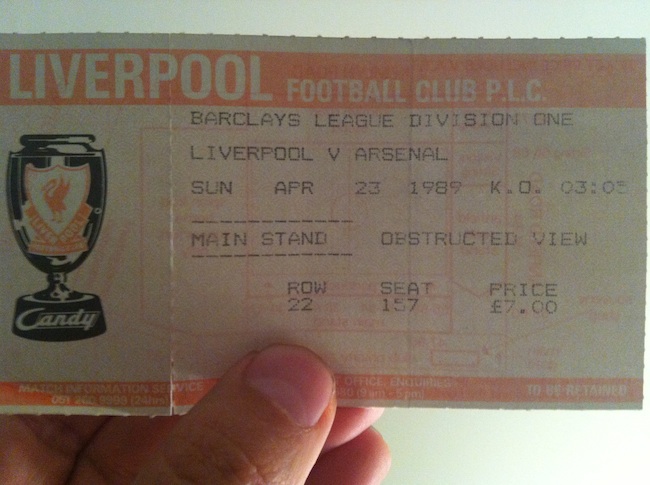This detailed photograph depicts a close-up of a vintage football ticket being held by a tan-skinned hand, with the thumb clearly visible. The ticket is primarily white, featuring bold orange stripes at both the top and bottom. The top stripe prominently displays in white capital letters "Liverpool Football Club, PLC." Below the top stripe, the ticket's main text in black reads: "Barclays League Division 1, Liverpool vs. Arsenal, Sunday, April 23, 1989, KO 3:05." The seating details specify "Main Stand Restricted View, Row 22, Seat 157," with a price of £7. On the left side of the ticket, there is an illustration of a black trophy with an orange crest or shield, possibly featuring a bird. The base of the trophy bears the word "Candy" in white letters.